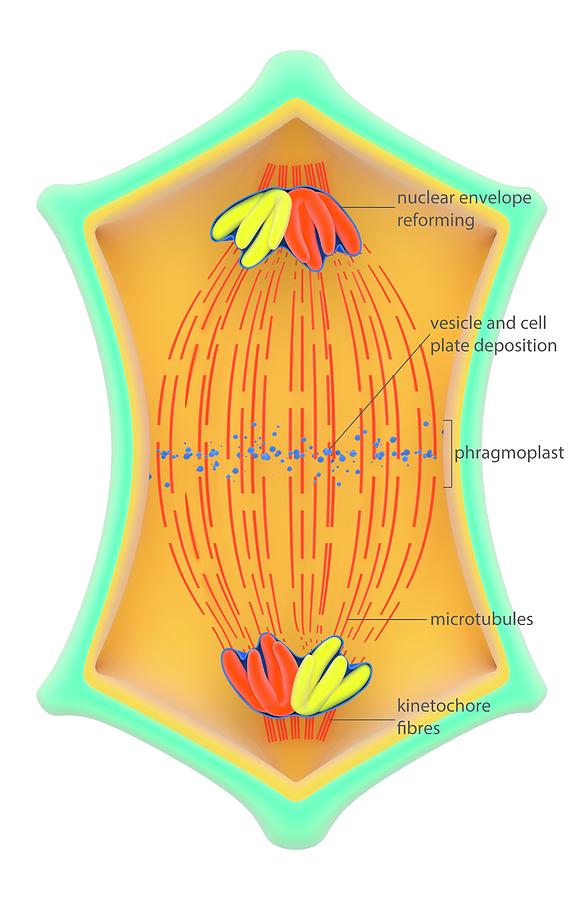The image is a detailed diagram of a cell, presented against a solid white background. The outline of the cell features a green border followed by a yellow border, with the cell's interior shaded in dark yellow. Prominent labels within the diagram point to various cellular components such as the nuclear envelope reforming, vesicle and cell plate deposition, phragmoplast, microtubules, and kinetochore fibers. Red lines and dashes traverse the diagram, accompanied by blue dots scattered across the center. At both the top and the bottom of the cell, red and yellow glands are depicted. The overall shape of the cell is compared to that of a partially inflated balloon, with an emphasis on the intricate network of components and their interconnections.